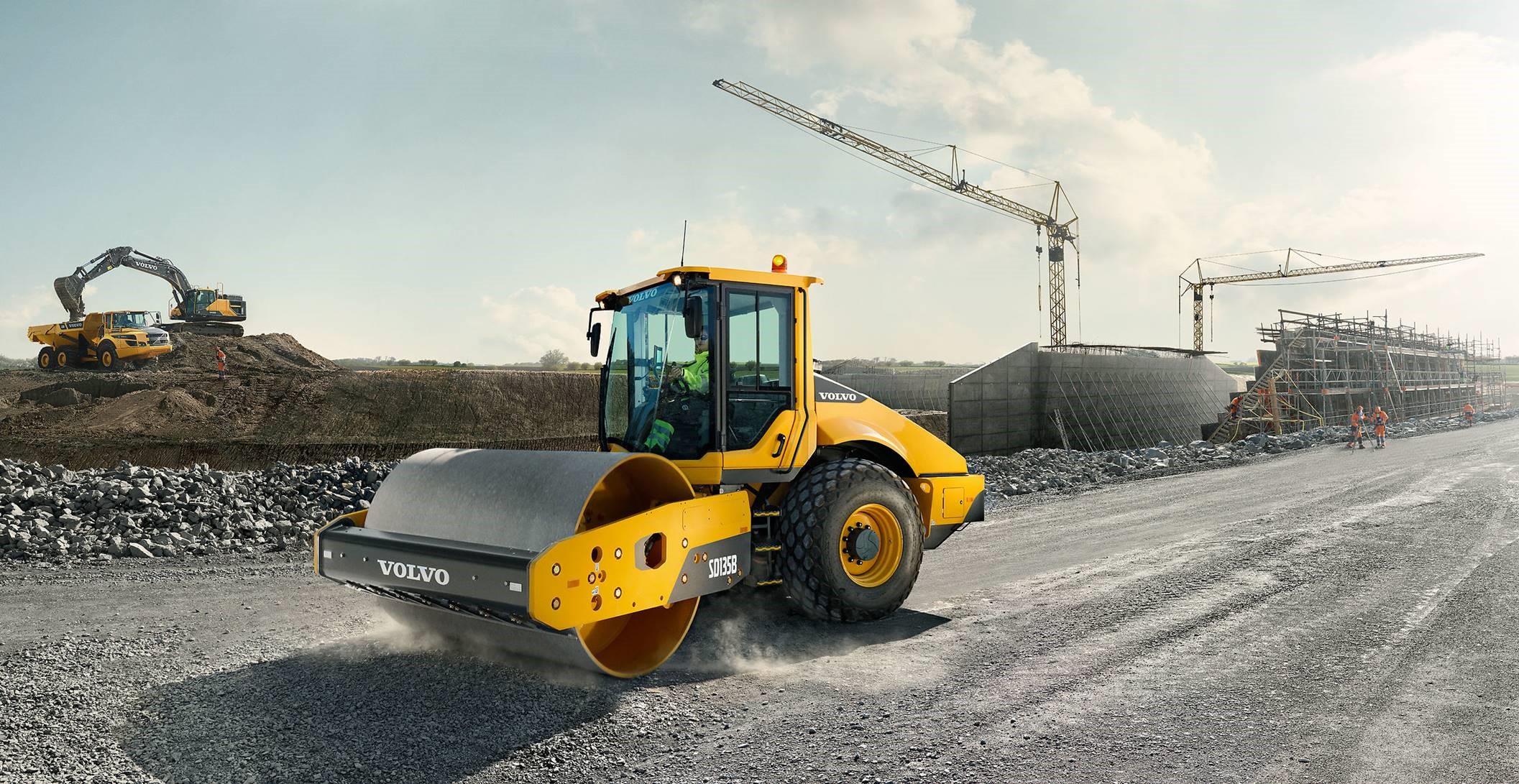This outdoor, full-color photograph captures a busy construction scene on a partly cloudy day. Dominating the foreground is a bright yellow and black Volvo steamroller, designed for flattening and compacting roads, driven by a person in a yellow vest. The steamroller is rolling over a gray, rocky road, with its massive front barrel clearly visible. Surrounding the Volvo roller, the construction site is bustling with activity. To the left, a bulldozer is seen pouring dirt into a red dump truck, while in the center right, two construction workers in safety orange stand by concrete forms set up as walls. The background features two large cranes and a dirt-covered hill. Further details include a backhoe and a Volvo dump truck being filled by an excavator. The top third of the image is filled with the sky and clouds, capturing the natural light of the day.